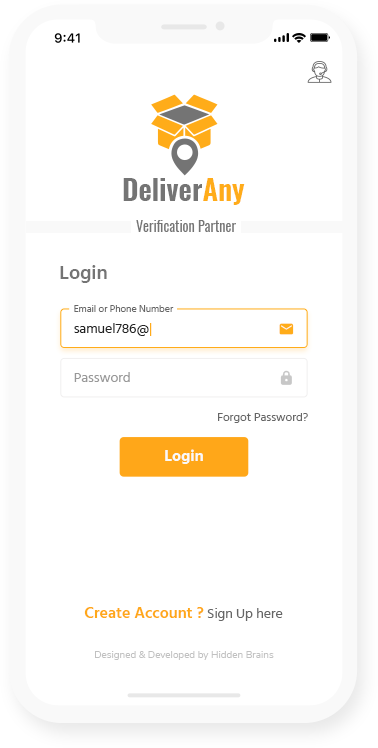The screen displays a smartphone interface with the time reading 9:41 AM and a fully charged battery indicator. The main focus is a login page for a service called "DeliverAny - Purification Partner." Users can log in by entering their email or phone number in a designated field, currently showing "Samuel786@". Below this, there is a blank password field. An orange 'Login' button sits prominently below the fields.

Additional options like 'Forgot Password' and 'Create Account' are available, allowing users to reset their password or sign up for a new account, respectively. The interface is designed with a color scheme of orange, gray, white, and light and dark gray, making it visually cohesive. Black text is used for contrast, particularly for system information and text labels.

Notably, there is an orange envelope icon next to the email field and a gray lock icon next to the password field, indicating the purpose of each input. An icon of a person wearing a headset is situated in the upper right corner, likely representing customer support. The footer mentions "Designed and Developed by Hidden Brains," giving credit to the creators of the interface. Above the "DeliverAny" logo, there is an orange box with a gray interior and open sides, adding a unique design element to the overall layout.